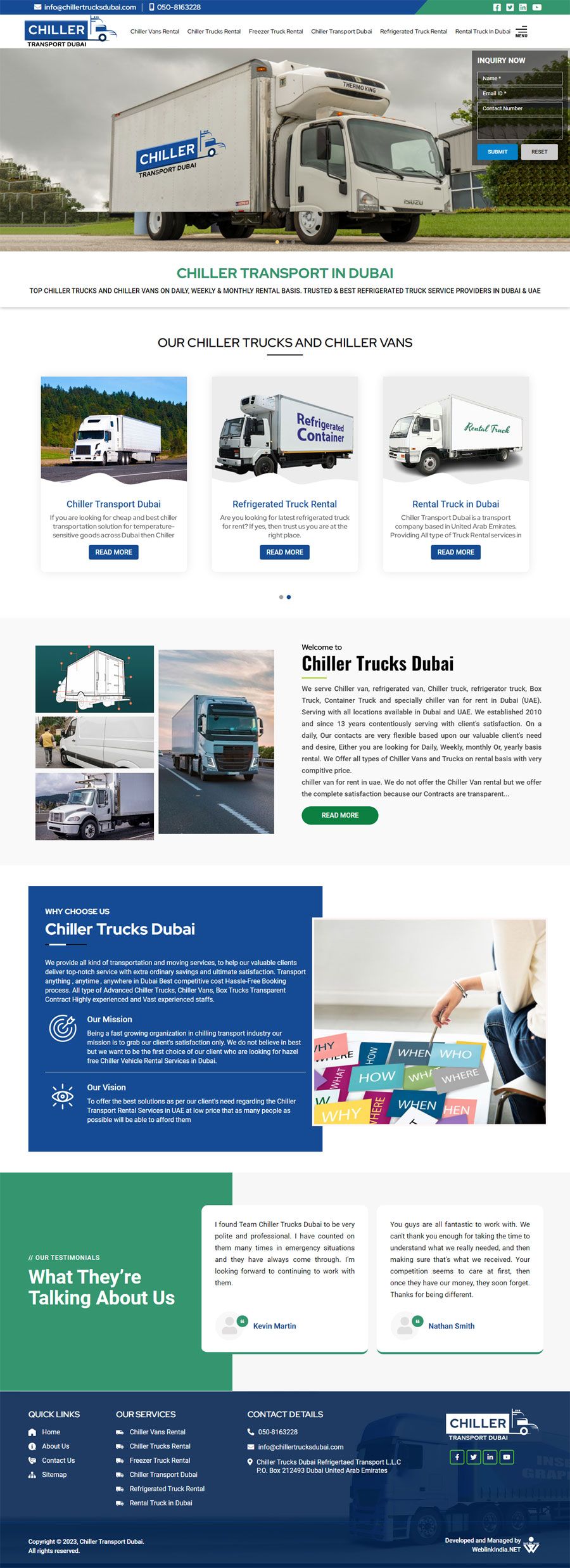Sure, here is a cleaned-up and detailed caption for the image:

---

The image features a blue background with white text. In the top right corner, the word "Chila" is prominently displayed. Positioned just below small and unreadable tabs at the top, there is an image of a truck facing towards the right. The truck's container also bears the word "Chila," matching the color of the logo.

Below the truck image, there's a green text that reads, "Chila Transport in Dubai." Additionally, the phrase "Our Chila Trucks and Chila Vans" appears below this. Three trucks are showcased beneath this text. The truck on the left is labelled "Chila Transport, Dubai," the middle truck reads "Retruck" with the subtitle "Retirement Truck Rental," and the truck on the right is labeled "Rental Truck in Dubai."

Further down, the same three trucks reappear with accompanying small and hard-to-read descriptions. On the bottom right, the text "Chila Trucks, Dubai" is visible. In the bottom left corner, against a blue background, there's a heading "Why choose us, Chila Trucks, Dubai?" followed by green text at the bottom that reads, "What they are talking about us and their reviews," though the reviews are blurry and difficult to read. At the very bottom, contact details, services, and quick links are listed on the left side.

---